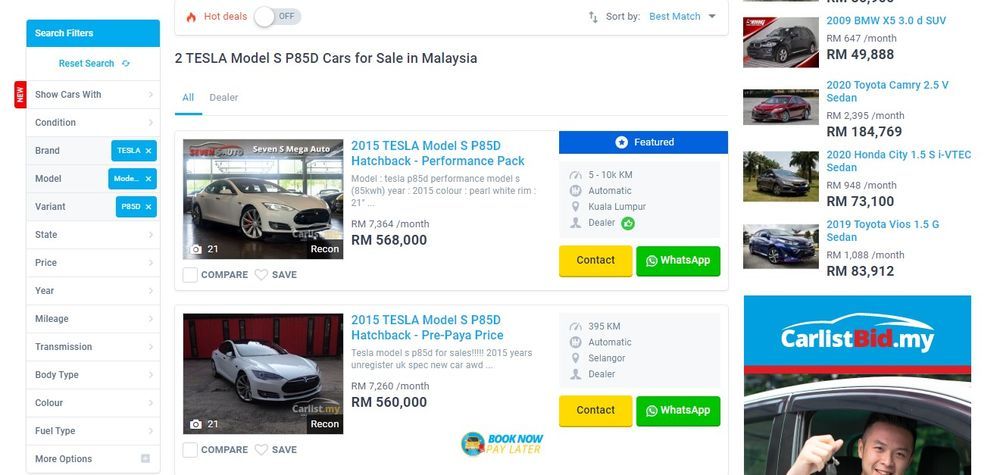In this rectangular screenshot, we are presented with an interface featuring a white background. Elliptical filters are positioned in a blue box at the upper left corner, reading from top to bottom: "Reset Search," "Show Cars With," "Condition," and "Brand." To the right of "Brand" is another blue box labeled "Tesla." Beneath this, the options continue with "Model," and next to it in a blue box is "Mode." Following this pattern, "Variant" appears with "P850" in a blue box to its right. Below these, there are additional categories: "State," "Price," "Year," "Body Type," "Color," and "Fuel Type." 

To the right of this list, in bold black text, it states, "Two Tesla Model S P85D cars for sale in Malaysia." The featured image showcases one of the cars – a gleaming white Tesla Model S P85D situated in a showroom. The description of the vehicle reads: "2015 Tesla Model S P85D Hatchback Performance Pack," highlighting the car’s model year and specific performance package.